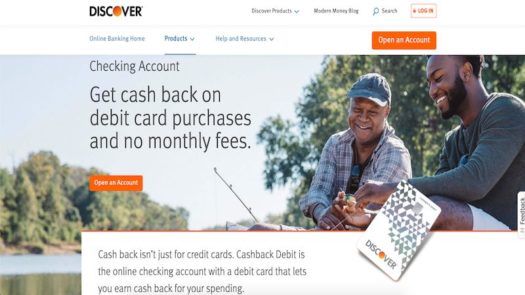The image features a clean, white background with the title "DISCOVER" prominently displayed in the top left corner. The word "DISCOVER" is highlighted with a yellow 'O,' while the other letters are in black. At the top right, there are several tabs labeled "DISCOVER," "PRODUCT," "REDEEM," and search and lock icons. The lock icon is in orange, whereas the rest of the tabs are in black. Right below the lock icon, there's an orange button labeled "OPEN ACCOUNT."

On the left side below the "DISCOVER" heading, there are several navigational tabs including "ONLINE BANKING," "HOME," "PRODUCT," "HELP AND RESOURCES," and "PRODUCTS," with "PRODUCTS" being highlighted.

In the main content area under the "PRODUCTS" tab, there is a section of text on the left side in black that reads: "CHECKING ACCOUNT, GET CASHBACK ON DEBIT CARD PURCHASES, and NO MONTHLY FEES." Below this text, there is an orange button that says "OPEN ACCOUNT."

On the right side of the image, there are two men fishing in a river, surrounded by trees and a blue sky in the background. At the bottom of the image, the text reads: "CASHBACK ISN'T JUST FOR VERTICAL CARDS. GET DEBIT IS THE ONLINE CHECKING ACCOUNT WITH A DEBIT CARD THAT LETS YOU EARN CASHBACK FOR YOUR SPENDING." This text is also in black against the white background.

Overall, the combination of intuitive navigation, promotional messages, and an inviting image suggests a seamless and rewarding online banking experience.